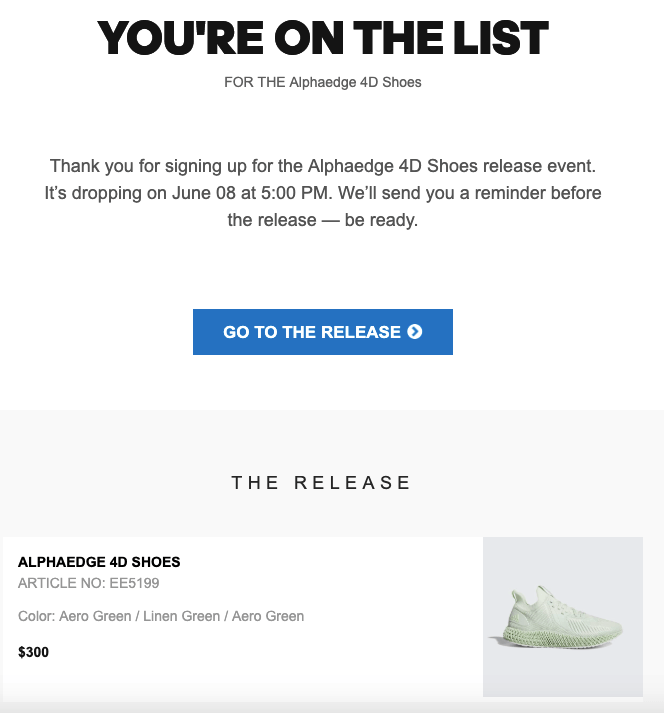**Detailed Caption:**

Displayed prominently at the top of the image is a large, bold, capitalized text reading "YOU'RE ON THE LIST." Beneath this headline, more detailed text announces, "for the Alpha Edge 40 shoes release event." This is followed by a larger note stating, "Thank you for signing up for the Alpha Edge 40 shoes release event." The text informs viewers that the release is scheduled for June 8th at 5 p.m., and reassures them that a reminder will be sent before the release, encouraging them to "Be ready."

Below this informational text, a large blue button with white typography serves as a call to action, reading "Go to the Release" with an arrow pointing to the right.

Following this section, there's a bold headline stating "Alpha Edge 40 shoes," accompanied by product specifics: "Article Number EE5199" and "Color: Arrow Green / Linen Green / Arrow Green." The price is listed as "$300."

To the right of this detailed product description is an image of the shoe itself. The Alpha Edge 40 appears to be a white running shoe, notable for its unique sole which seems 3D-printed. The cushioning part is composed of a grid interlace of support lines rather than a traditional solid foam. The shoe is set against a light gray background.

Below this shoe image is a peach-colored bar extending the full width of the site, all set against a clean, white background.